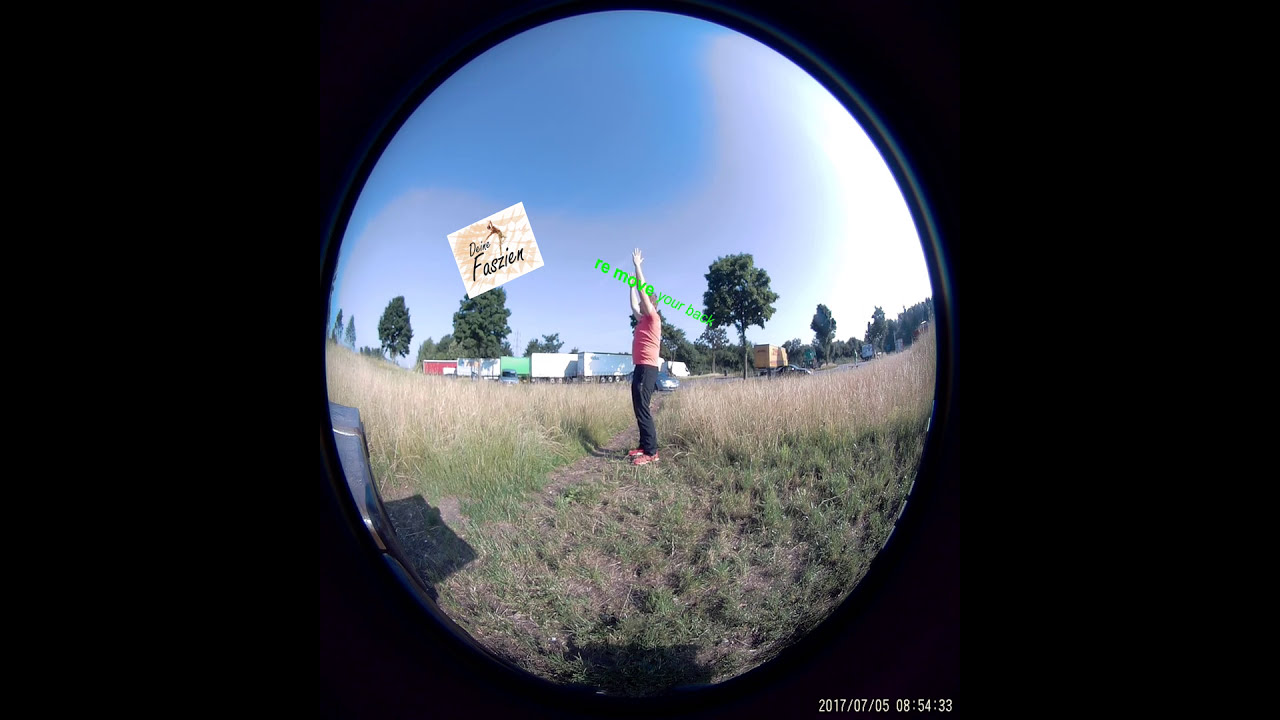In this fishbowl-like image, we see a convex mirror capturing a person standing in an overgrown, somewhat dying grassy field. The individual is dressed in a short-sleeved pink t-shirt, dark jeans or pants, and pink sneakers, and they have their arms raised, appearing to hold a kite or a sign, which is yellow and white with black lettering that is too distant to decipher clearly. Additionally, a name tag that seems to say "Dan Fazian" is affixed to their shirt. The background features large green trees and several trailer trucks, set against a sky that is mostly clear with a few large white puffy clouds. There's also a green sign with the words "remove your back," contributing to the scene's intriguing details.